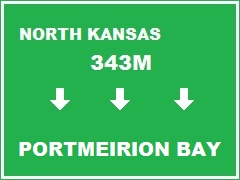This high-quality, computer-generated image features a green road sign with comprehensive details. At the top of the sign, in bold white letters, it reads "North Kansas." Below this, "343 M" is prominently displayed, indicating a distance measurement of 343 meters. Directly beneath the distance marker, three downward-pointing arrows are aligned horizontally with a slight gap between each. At the bottom of the sign, the destination "Portmeirion Bay" is clearly written. The bright green sign is accentuated by a thin white border and is further framed by a broader green border, enhancing its visibility and readability.